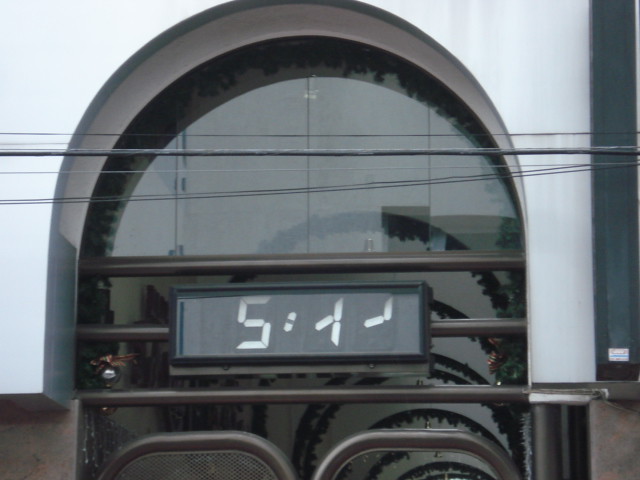The image showcases the entrance to an unidentified building, possibly commercial. It features a prominent white arch structure framing a multi-pane window with crossbars filling the entire space within the arch. At the bottom, partially visible, are the tops of what appear to be two doorways, outlined with black piping. Mounted on a horizontal pipe across the archway is a black rectangular clock with a white segmented display. The display clearly shows the digit '5' followed by a colon, but the subsequent two characters are not recognizable numbers. The first of these characters consists of an upright segment on the right side with a 45-degree crossbar, resembling a distorted or incomplete numeral one. The final character includes one upright segment at the top right and a diagonal segment connected to it, forming an unidentifiable figure. This discrepancy, especially with the presence of the correct numeral five and colon, creates a confusing visual anomaly, as the unrecognizable characters do not align with standard Arabic numerals typically seen on such displays.